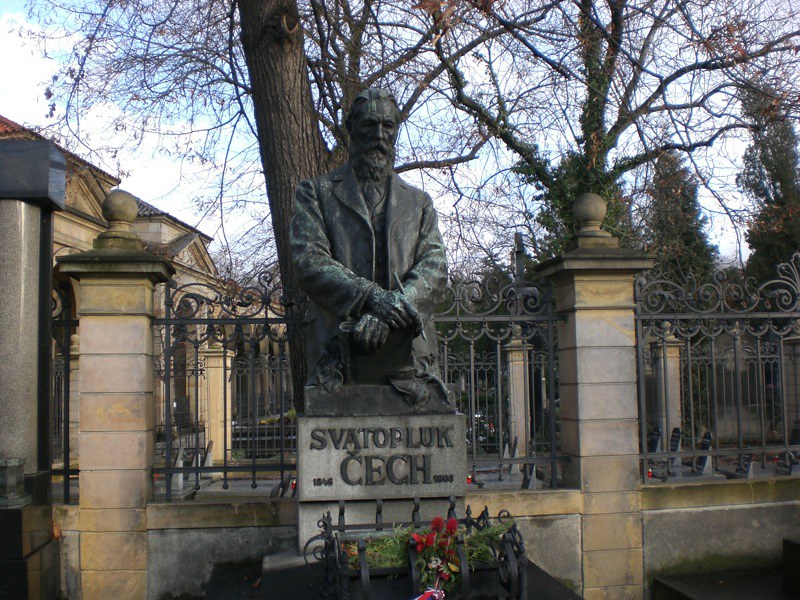The image showcases a statue of a bearded man with folded arms, made of dark gray material, either stone or metal. It prominently features the name "Svatopluk Čech" inscribed at its base, along with the years 1846 to 1903. The statue is seated on a stone-like base with black lettering and is positioned in a cemetery setting. In the foreground, there are plants and flowers adorning the base of the statue. Surrounding the statue are faded, yellow-tinged columns and a large wrought iron gate supported by concrete columns. The background reveals a mausoleum and leafless trees, suggesting it's late in the year. The sky above is light blue with puffy white clouds, indicating daytime. The scene includes a very ornate gray fence and two shorter white pillars with gold knobs adjacent to the statue. The architecture and ambiance suggest a European town, possibly Czechoslovakia.